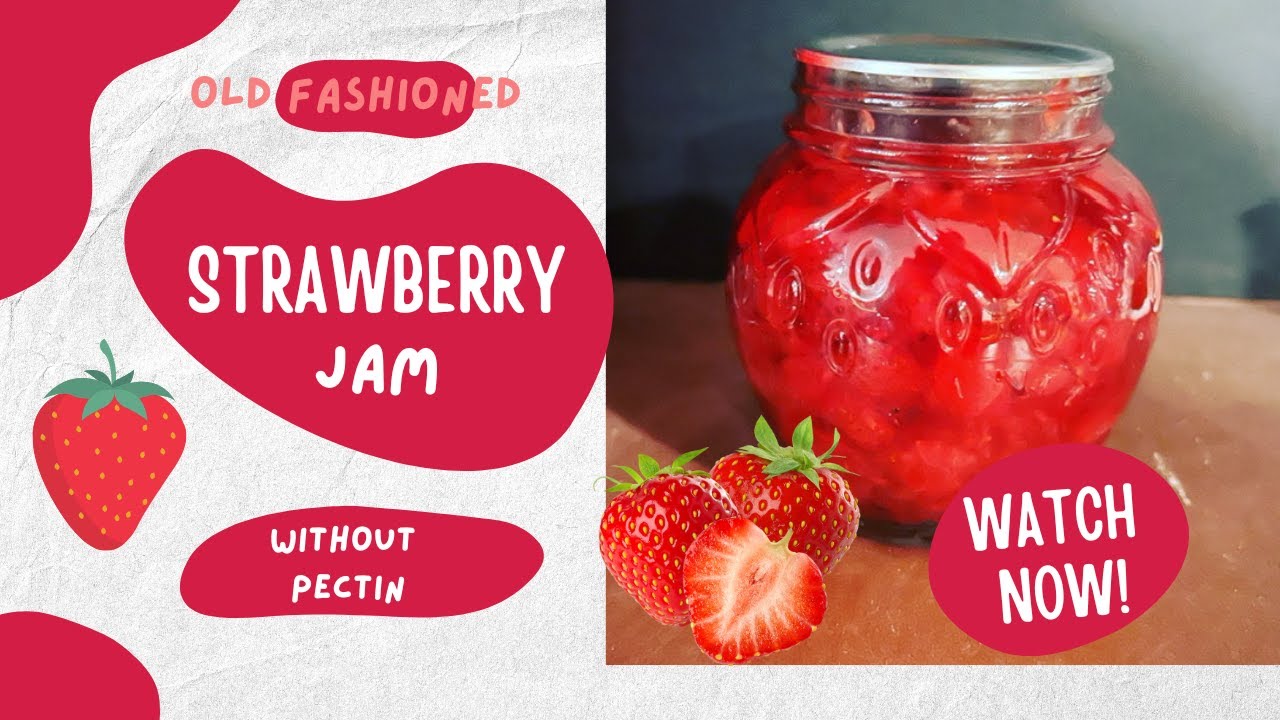The advertisement features a rectangular image wider than it is tall, showcasing an old-fashioned strawberry jam without pectin. The centerpiece is a clear glass jar of strawberry jam with a silver screw-on lid, set on a brown or tan table. The background is a gray wall illuminated with soft white light, containing hints of texture and red patches. To the left of the jar, a circle with the text "Watch Now!" stands out. Accompanying the central image, there's a drawing of a strawberry and an array of three strawberries, one of which is cut in half to reveal the interior. The entire setup is framed by a white and red background, creating a visually appealing and nostalgic advertisement.